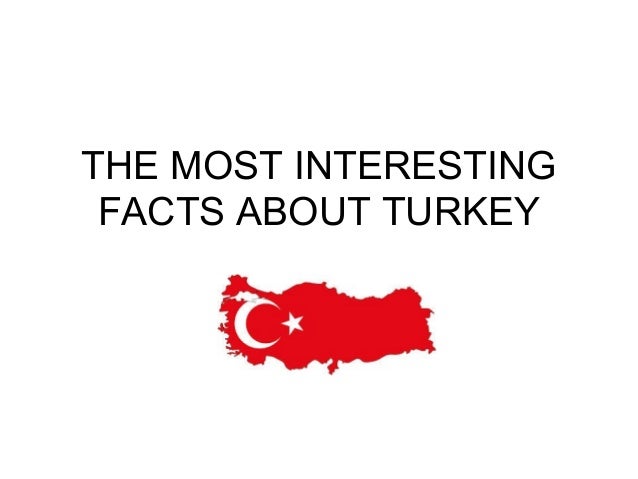The image features the outline of Turkey prominently centered against a white background. The entire shape of the country is filled with a solid red color. On the left side of the red area, there is a large white crescent moon, and next to it on the right, there is a white five-pointed star. Above the outlined map of Turkey are two lines of text in black Arial font, all capitalized letters, reading "THE MOST INTERESTING FACTS ABOUT TURKEY." The text is also centered, directly positioned above the red outline of the country. The simplicity of the background highlights the striking use of black, white, and red colors to draw attention to the map and the caption.